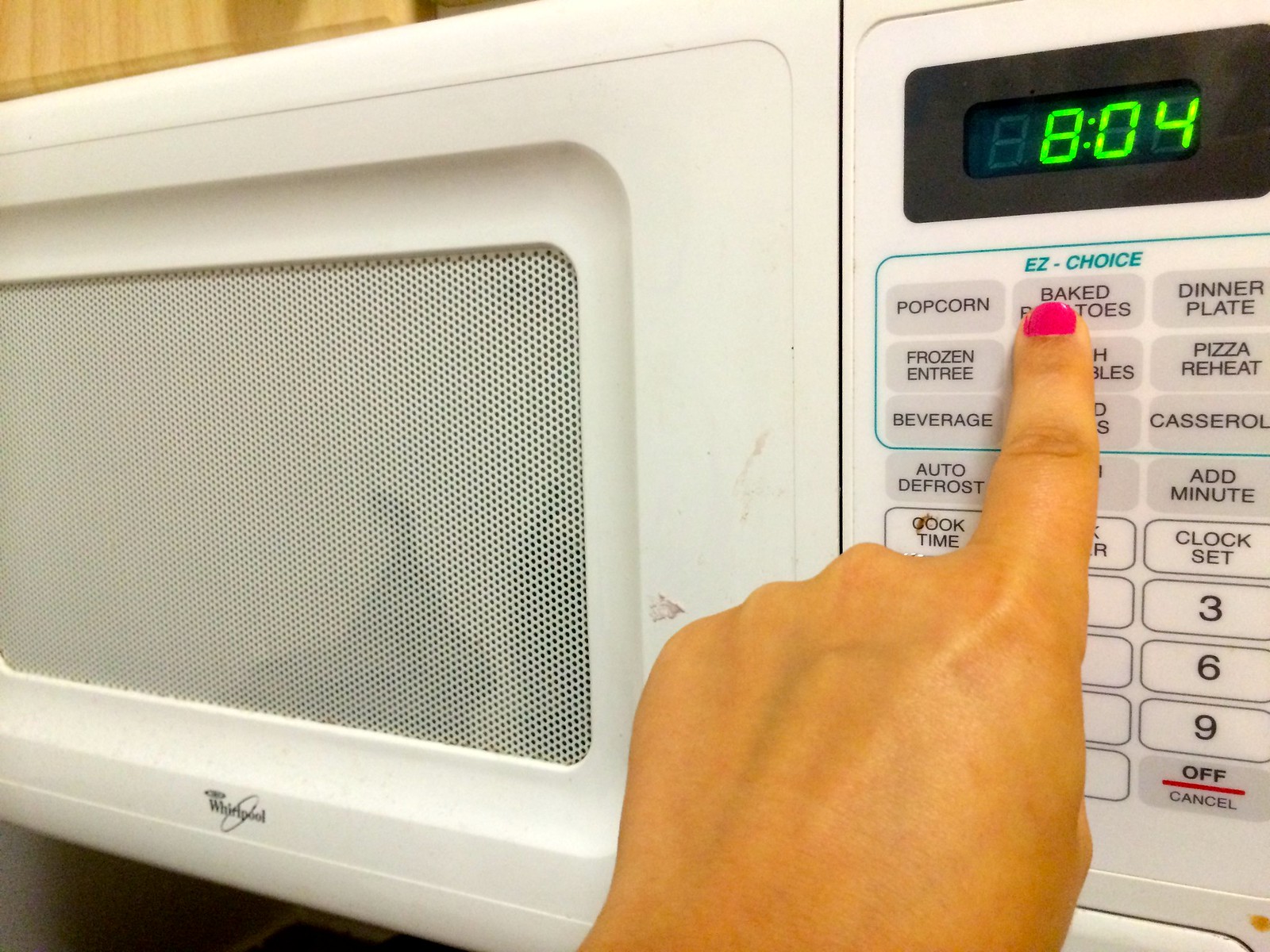The image depicts a woman using a white Whirlpool microwave, which appears to be mounted underneath a cabinet with light wood tones. The microwave looks quite old and has some scratches and a bit of dirt on it. The woman’s hand, with a bright pink nail polish on her index finger, is poised to press the "Baked Potatoes" button from the "Easy Choice" menu, which is labeled in a seafoam green color. The "Easy Choice" menu includes options like popcorn, baked potatoes, dinner plate, frozen entrée, frozen vegetables, pizza reheat, beverage, and casserole. The microwave’s display screen shows the time "8:04" in green. The microwave door, shut during the photo, has a window with small black perforations.